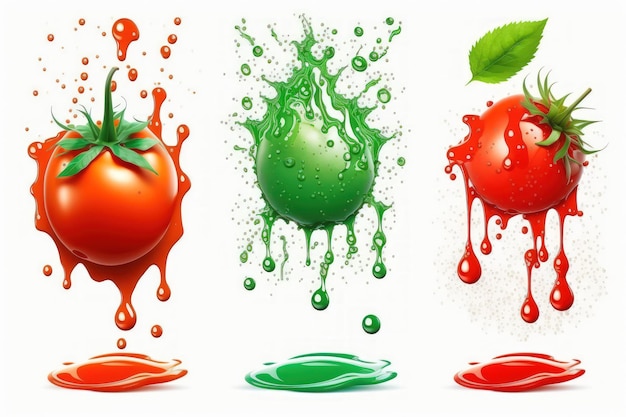This artwork is a three-panel series set against an off-white, light cream-colored background. The left panel showcases a detailed red tomato with a stem, splattered against the backdrop with vibrant red liquid dripping down, forming a red puddle beneath it. Drops can be seen flying upwards and leaking downwards from the impact. The middle panel features a green tomato, also stemless, which appears to have splashed green juice explosively, creating a dynamic spread of green droplets around it and a pooling of green liquid at the bottom. In the right panel, another red tomato with a noticeable green stem and stalk at the two o'clock position is depicted, accompanied by a jagged-edged leaf positioned above it, although the leaf is not from a tomato plant. Similar to the first panel, this tomato is surrounded by splatters of red liquid cascading downwards into a red puddle on the ground. Each panel captures the essence of the fruit hitting the wall with liquid splattering and pooling in corresponding colors.